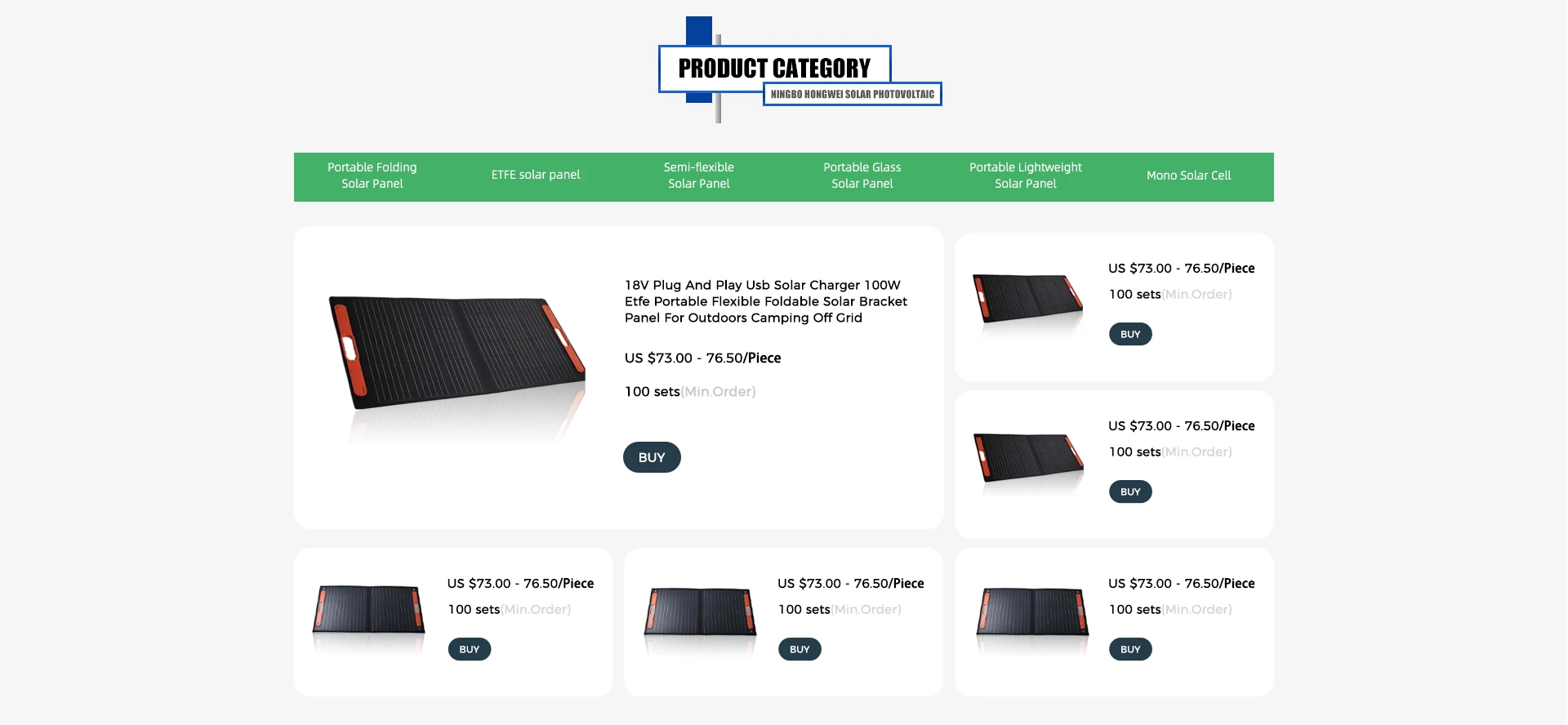In this image, we see a screenshot featuring a light gray background. At the very top center of the screenshot, the website's name is prominently displayed as "Product Category" in bold black text outlined in blue, accompanied by a logo consisting of a blue rectangle with a gray bar to its right. Directly beneath this, in smaller, gray text, it reads "Ningbo Honggui Solar Photovoltaic". 

Below this heading, there is a green horizontal banner listing various product categories from left to right: "Portable Folding Solar Panel, ETFE Solar Panel, Semi-Flexible Solar Panel, Portable Glass Solar Panel, Portable Lightweight Solar Panel, and Mono Solar Panel". 

Each mentioned category is visually represented below the banner by detailed photo images of the respective solar panels. In the top right section of the image, there is a black panel with a price range indicated as "U.S. $73 through $76.50 per piece". 

Additionally, next to the image of the black panel, there is a black action button labeled "Buy" for user interaction.